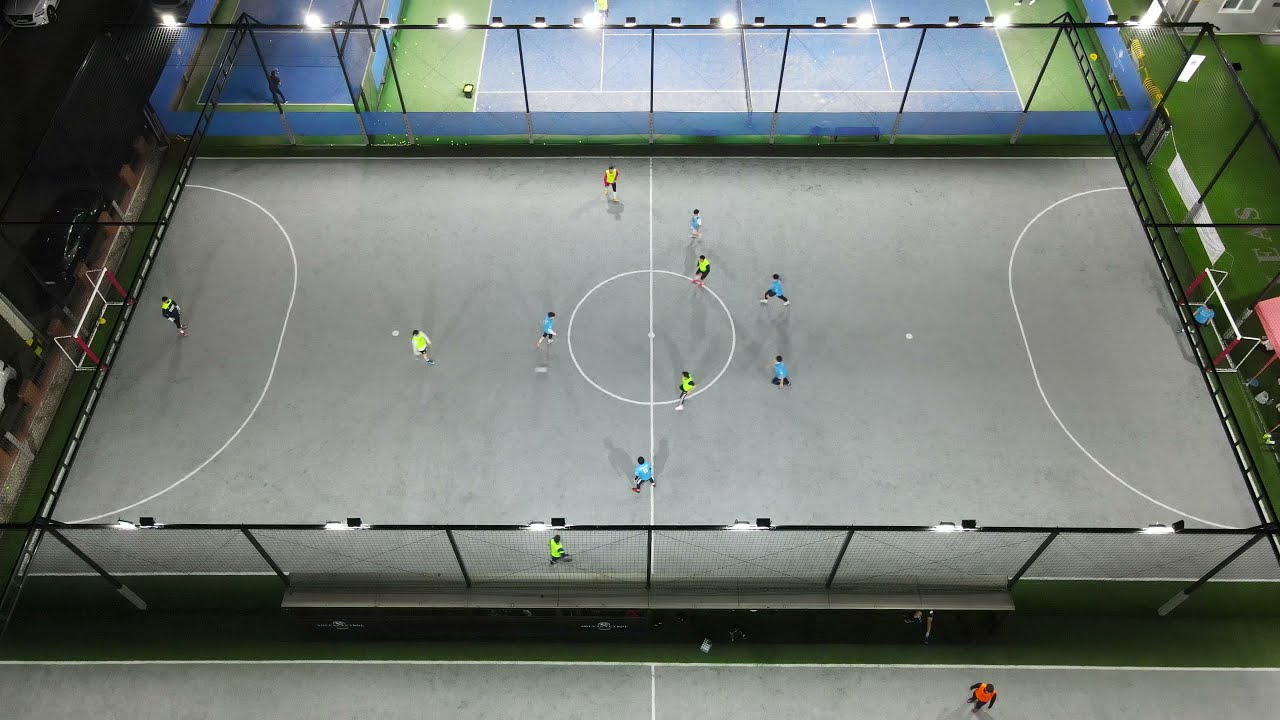The image is an aerial view of a sports facility featuring a large, concrete court that resembles a basketball court but is likely set up for an indoor soccer or handball game. The court is surrounded by a chain-link fence, and there are fluorescent lights mounted on top of the fence, illuminating the playing area. Adjacent to the main court, a tennis court can be seen. 

On the court, two teams are engaged in a match, each comprising five players—four outfield players and one goalie per team. One team is dressed in neon yellow jerseys, while the opposing team wears lighter blue jerseys. The ball is positioned near the center, marked by a circle with a line through it, and additional lines demarcate the goal areas.

Outside the fenced court, a person wearing an orange or red vest is visible, possibly a coach or a spectator. There is also a patch of green on the right side outside the fence. The image captures the dynamic scene from above, providing a comprehensive view of the ongoing game and the surrounding facility.